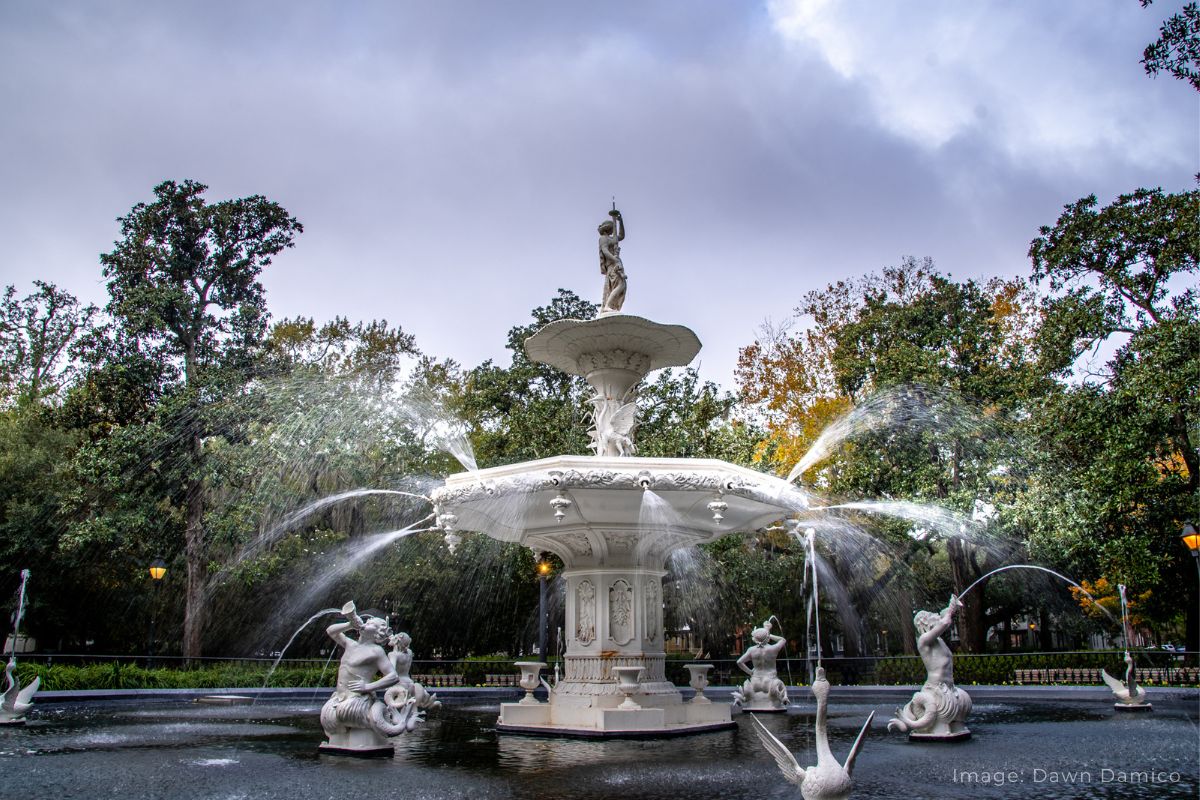The photograph captures a large, intricately designed Roman-style fountain located in a park during mid-afternoon. The sky above is a grayish blue with patches of wispy clouds and a prominent white cloud in the upper right-hand corner. The fountain itself is grand, with a pale white to cream color and composed of multiple tiers. At its broad base, statues of cherubs and ducks spew water, creating ripples and splashes in the surrounding pool. These figures encircle a large basin from which a tower-like structure emerges. This tower features another basin with water spraying from several points. Above, a cone element leads to the fountain's top tier, which holds a statue of a human figure draped in Roman attire, holding a stick in the air. The background includes a variety of trees of different heights and park lights that are turned on. The bottom right corner of the image displays the text "Image Don D'Amico."